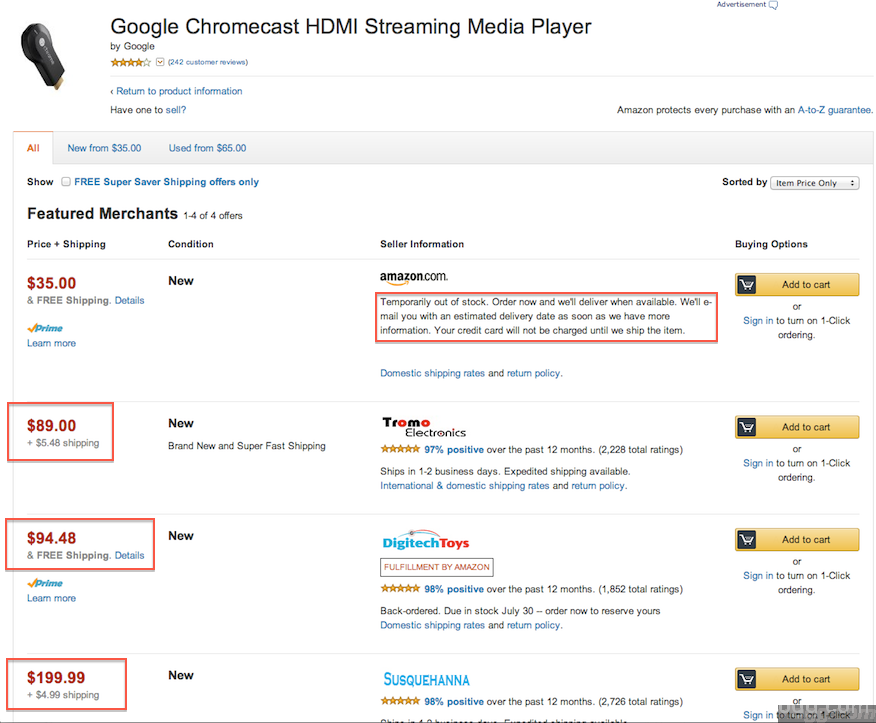**Low-Resolution Screenshot of Amazon Seller Page for Google Chromecast HDMI Streaming Player**

The image is a low-resolution screenshot of an Amazon seller information page for a Google Chromecast HDMI streaming player. The dominant background color is white, with clickable blue text links. Yellow "Add to Cart" buttons are prominently displayed, featuring black text and a small black and white shopping cart icon on the left side of each button.

The main item being sold is a Google Chromecast HDMI streaming player by Google, identifiable by its tiny dongle design that plugs directly into the HDMI port of a display. Below the product description, a yellow star rating is visible.

The screenshot showcases three menu options at the top: "All" (which is the selected and highlighted tab), "New from $35," and "Used from $65 or $85" (the exact price is unclear due to the low resolution). Below these tabs, the text "Featured Merchants" is displayed in black.

The page lists four merchants, with Amazon.com at the top, offering the product for $35 but marked as out-of-stock. This status is encased in a red-outlined box. Other merchant listings show significantly higher prices: $89, $94, and $199.99, each highlighted within red squares, indicating their greater expense.